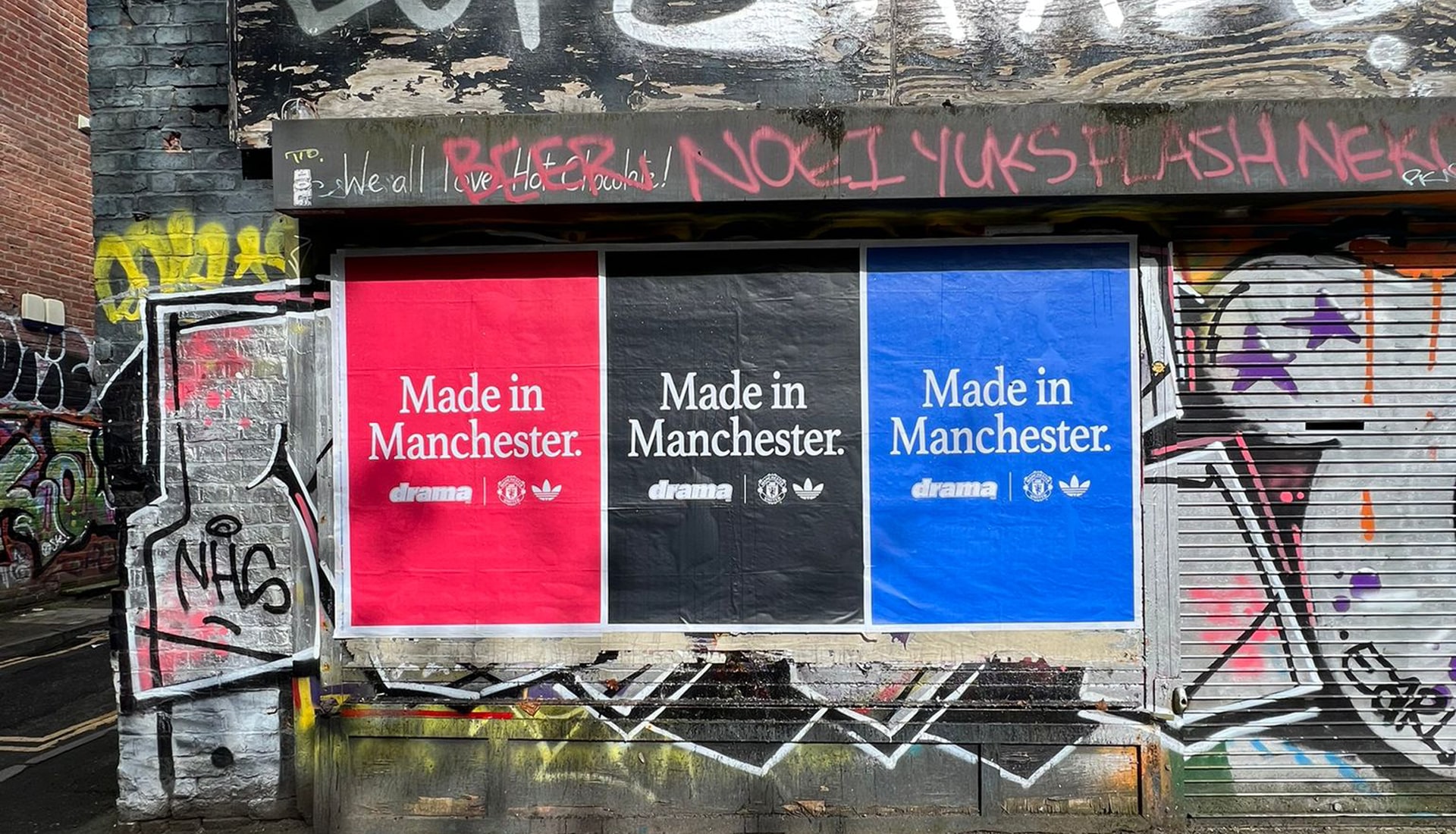This photograph features the side of a rundown storefront, characterized by its lowered metal gates and extensive graffiti. The storefront appears abandoned, with a metal grating on the right, typically used to secure the entrance, fully drawn down. The left portion of the storefront and its overhanging structure are heavily covered in various tags and street art, obscuring the original color of the building. Prominently displayed on the metal gate are three distinct posters, each bearing the phrase "Made in Manchester" centered in white text. These posters are side-by-side with thin white borders between them and have different background colors: red, black, and blue. Additionally, each poster includes the word "Drama" beneath the main text alongside two logos, one of which is identified as Adidas. The graffiti around the area includes legible tags such as "Earl," "NHS," and seemingly random letters and phrases like "beer," "noei," "yuks," and "flashneki." The bottom left part of the building opposite to this one, visible across a street or alley, is made of natural red brick and also shows signs of tagging, particularly on its lower section. The entire scene suggests a neglected area, with the imagery of the posters adding a contrasting pop of structured commercialism amidst the chaotic street art. Purple stars and other symbols adorn the graffiti-covered right section, enhancing the visual clutter.